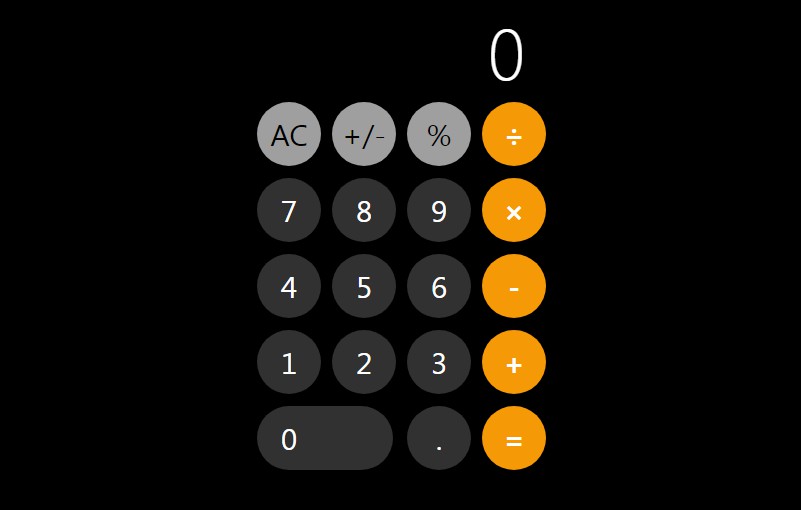The screenshot appears to be from a calculator app with a sleek, minimalist design. The interface has a predominantly black background at the top, highlighted by a large white "0" indicating the current value or result display. 

Beneath the display, there are five rows of buttons arranged in a 4x5 grid, except for the bottom row which contains three buttons. 

- The first row features three small gray circular buttons labeled "AC" (All Clear), a plus-minus symbol ("±"), and a percentage sign ("%"), followed by a yellow circular button with a division symbol ("÷").
 
- The second row consists of gray circular buttons with numbers "7", "8", and "9". Adjacent to these is an orange circular button displaying a multiplication symbol ("×").

- The third row continues with gray circular buttons for the numbers "4", "5", and "6", and an orange circular button with a minus sign ("−") at the end.

- In the fourth row, gray circular buttons for numbers "1", "2", and "3" are present, next to an orange circular button featuring a plus sign ("+").

- The fifth and final row includes a wider gray button with the number "0" (occupying the space of two typical buttons), a gray circular button with a period (".") for decimal points, and an orange circular button with an equals sign ("=") to execute calculations.

Overall, the app's design uses a consistent color scheme and geometric shapes to clearly differentiate between various functions and numerals, facilitating easy and intuitive use.